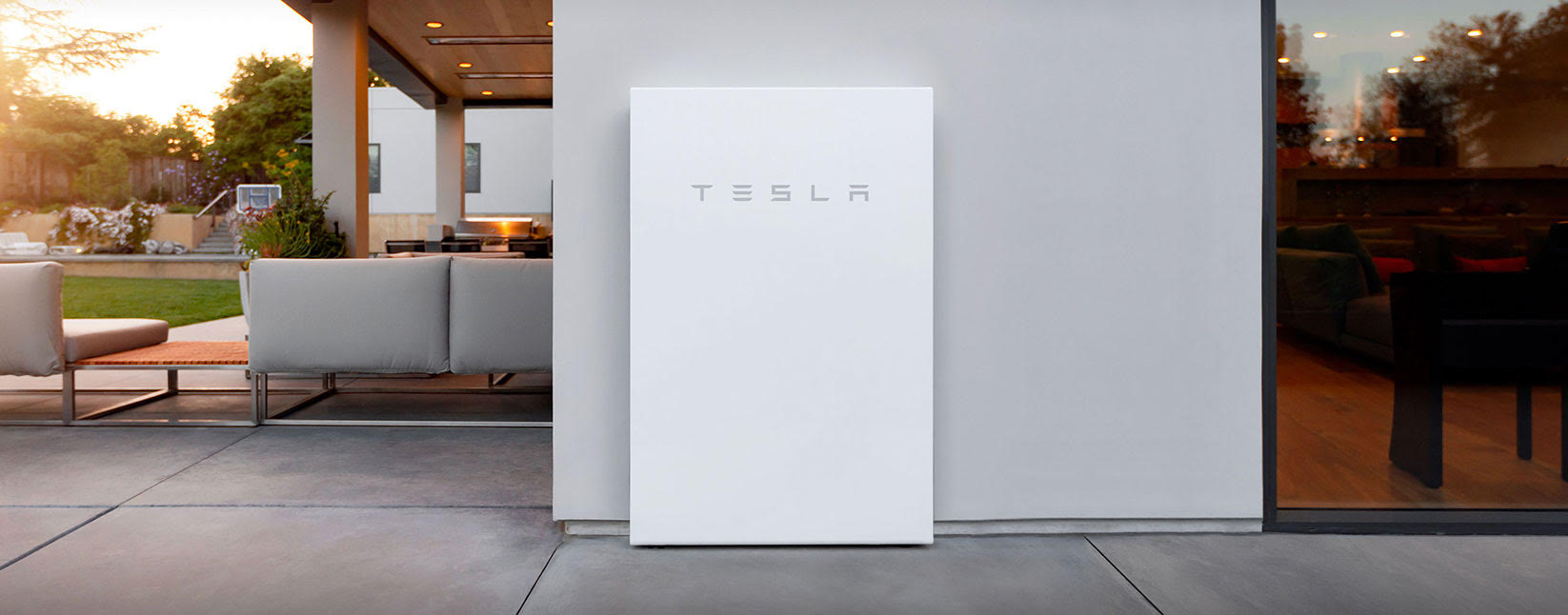A photograph captures a serene outdoor setting featuring a rectangular sign inscribed with "Tesla." The sign stands prominently in the foreground, while the background reveals a meticulously designed outdoor seating area. The ground is paved with aesthetically pleasing concrete squares, enhancing the overall elegance. 

On the right side of the image, illuminated windows of a building cast a warm glow, hinting at activity inside, while also reflecting parts of the exterior scene. The building's facade is painted a clean white, complementing the modern design ethos.

Beyond the seating area, a lush, green lawn stretches out, bordered by trees and possibly another residential structure or a garage. The distant view even includes a basketball hoop. Further adding to the ambiance, recessed lights are mounted on the walls, casting a gentle downlight that accentuates the tranquil evening atmosphere.